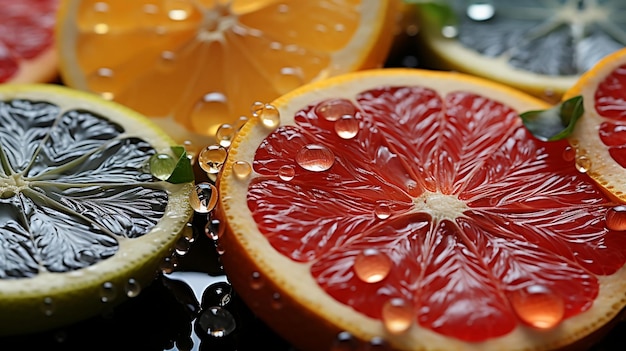The image features an array of fresh and vibrant citrus fruit slices arranged artistically. Prominently displayed in the foreground are slices of grapefruit, lime, and orange. The grapefruit slice is the most visible on the right, while a lime slice appears on the left. Behind them, slightly out of focus, are additional slices of either orange or lemon, contributing to the depth of the scene. Tiny green leaves, potentially mint, add a touch of greenery, with one leaf resting on the orange slice and another on the lime. The fruit slices are adorned with glistening water droplets, enhancing their fresh, juicy appearance. The backdrop features a dark area where a small pool of water seems to be collecting, adding to the overall refreshing and artistic appeal of the image.